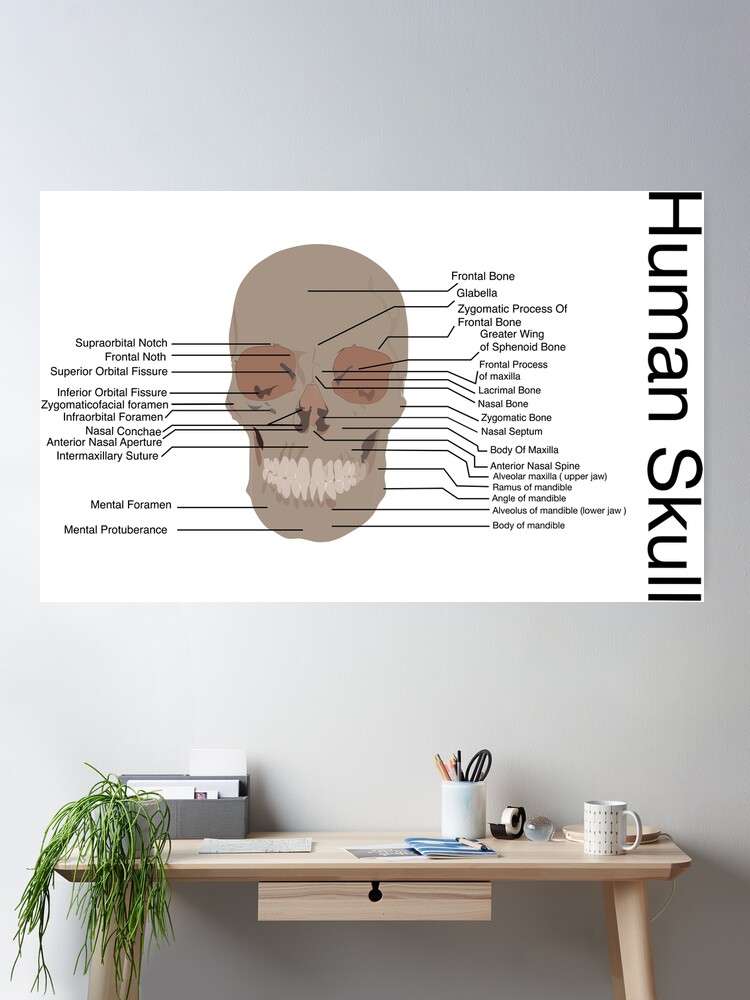The image showcases a small, light wooden desk situated against a gradient gray wall, which transitions from light gray on the right to a slightly darker shade on the left. Prominently above the desk hangs a rectangular educational poster featuring a detailed illustration of a brown and tan human skull. Numerous lines radiate from various parts of the skull to descriptive labels with text, though the print is too small to be legible. Along the right edge of the poster, the words "human skull" are printed vertically. The desk itself is neatly arranged with a variety of items: on the left, a leafy plant cascades over the edge, accompanied by a gray card holder, scattered papers, and a small book. Central to the desk is an organization of office supplies, including a pencil holder brimming with pens, pencils, and a pair of scissors, a clear tape dispenser, and a spherical glass object. On the far right sits a white coffee cup and an adjustable desk lamp, completing the tidy workspace.